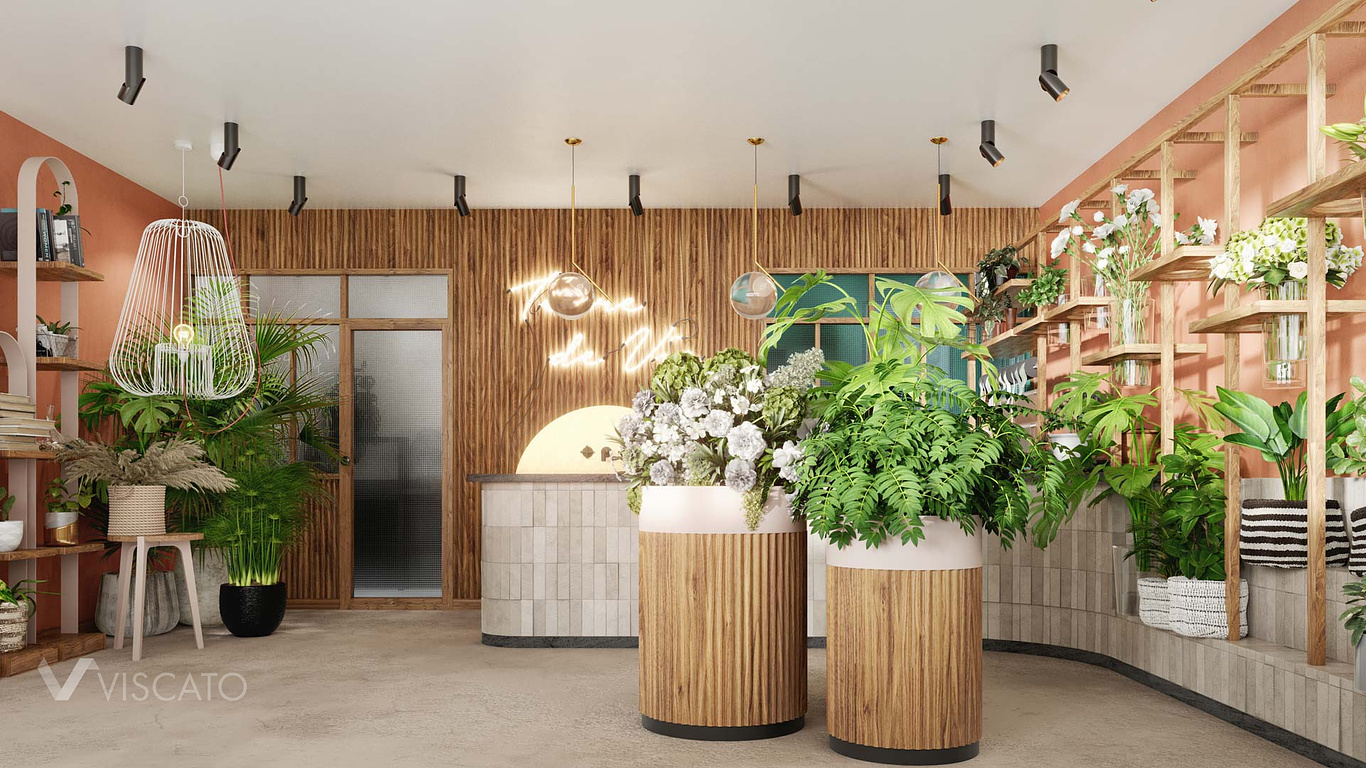This image depicts a beautifully designed indoor space, likely a lobby or lounge area of a massage studio or beauty parlor, showcasing a minimalist aesthetic with an abundance of greenery. The room features a stunning combination of light grayish beige flooring and walls painted in a light salmon pink. Dominating the center of the room are two large freestanding wooden planters; one brimming with lush green ferns and the other displaying a vibrant floral arrangement. Behind these planters is a back wall paneled with thin strips of wood, giving the room a tropical feel.

A sweeping stone or tile countertop extends from the center to the right-hand side of the room. Above it hang spherical glass chandeliers and a distinctive light fixture resembling a birdcage, adding a touch of elegance and charm. The right wall is adorned with several wooden shelves, each overflowing with various plants and flowers in different pots, creating a lively and fresh ambience.

The left side of the room features another set of wooden shelves with books and additional plants, and the bottom left corner prominently displays a large "V" along with the word "Viscato." The back wall also includes a glass door with windows, allowing natural light to pour in and further brighten the space. Black can lights are strategically placed to illuminate the wooden walls, while transparent globes hanging from the ceiling enhance the room's inviting atmosphere. Additionally, there is signage in bright lighting spelling "DeVille," contributing to the room's stylish and serene vibe.